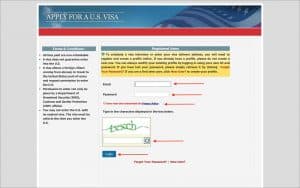The image depicts a small and somewhat unclear screenshot of a standard white webpage layout. At the top, there is a blue banner featuring an American flag on its right side, followed by a red bar below it. The primary section of the webpage contains a white background with text throughout. On the left, there is a narrow column with a small blue banner and some text that appears to be in reverse, while the right column features another small blue banner along with a yellow section. Below these areas, it includes fields designed for user interaction, such as input fields for a username and password, and a CAPTCHA verification section to confirm the user is human. The small size of the image makes it challenging to parse fine details and text.